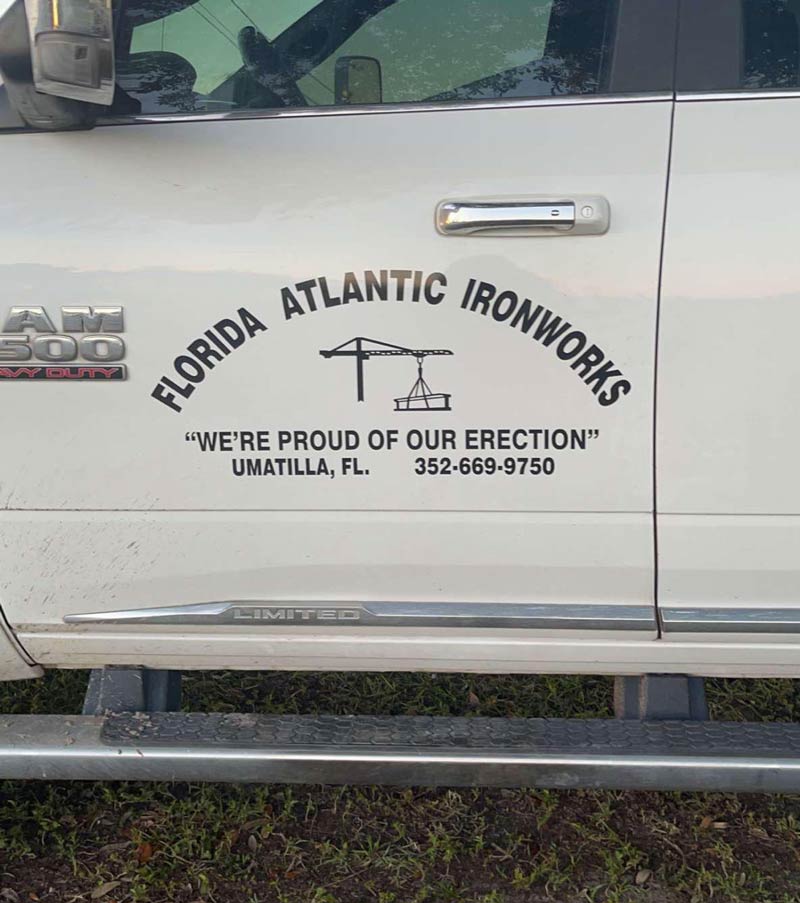The image reveals the exterior of a white Dodge Ram truck, specifically focusing on the left-hand driver's side door. At the top of the image, the partial window and side mirror are visible, while a silver door handle gleams against the white vehicle. The grey and silver step-up into the truck is also noticeable.

The main portion of the image showcases business advertisements in black text on the white door. At the top, the business name "Florida Atlantic Iron Works" appears in an arch, accompanied by a graphic of a crane lifting a steel girder. Beneath the business name, the slogan "We're proud of our erection" is displayed, followed by the location "Umatilla, FL" and a phone number, 352-669-9750. The lower part of the image shows the truck parked on a patch of grass and dirt.